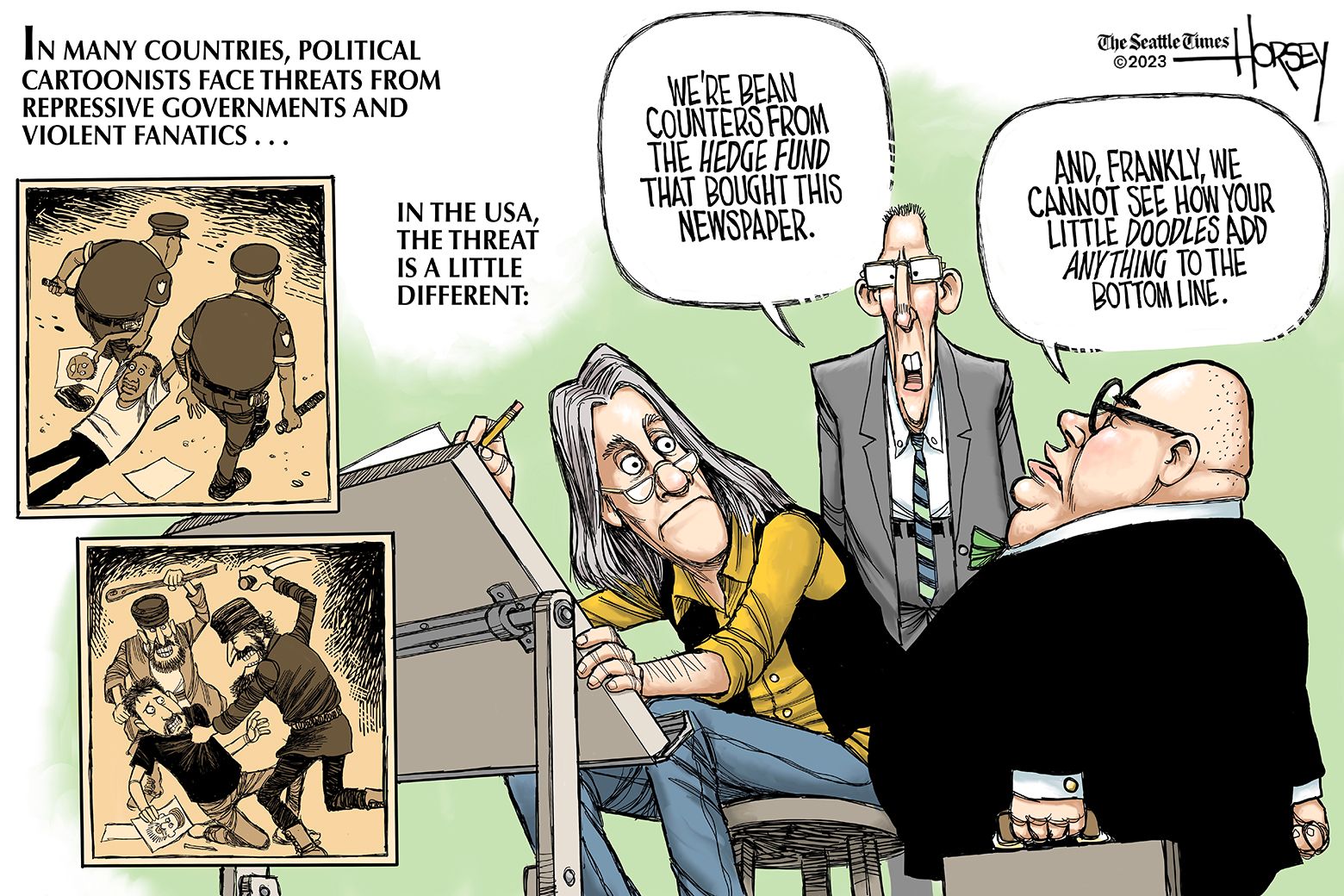This detailed political cartoon from the Seattle Times, illustrated by Horsey in 2023, juxtaposes the varied threats faced by political cartoonists around the world. The upper left corner features an introductory text stating, "In many countries, political cartoonists face threats from repressive governments and violent fanatics." This is illustrated by two inset images: one depicts a cartoonist being violently dragged away by two police officers wielding billy clubs, while the other shows a cartoonist being savagely beaten by two attackers, one armed with a club and the other with a knife. This grim portrayal contrasts starkly with the main image, which presents a different kind of threat faced by cartoonists in the USA. Here, an older cartoonist with long gray hair, glasses, a yellow shirt, a black vest, and blue jeans is diligently working at his angled drawing table. Behind him stand two corporate figures dressed in suits. One, with square glasses and a gray suit, declares, "We're bean counters from the hedge fund that bought this newspaper." The other, a shorter, obese man with round black-framed glasses and carrying a suitcase, adds, "And frankly, we cannot see how your little doodles add anything to the bottom line." While not subjected to physical violence, the American cartoonist's livelihood is threatened by the financial priorities of the newspaper's new owners, highlighting a subtler yet significant danger to the freedom of expression.